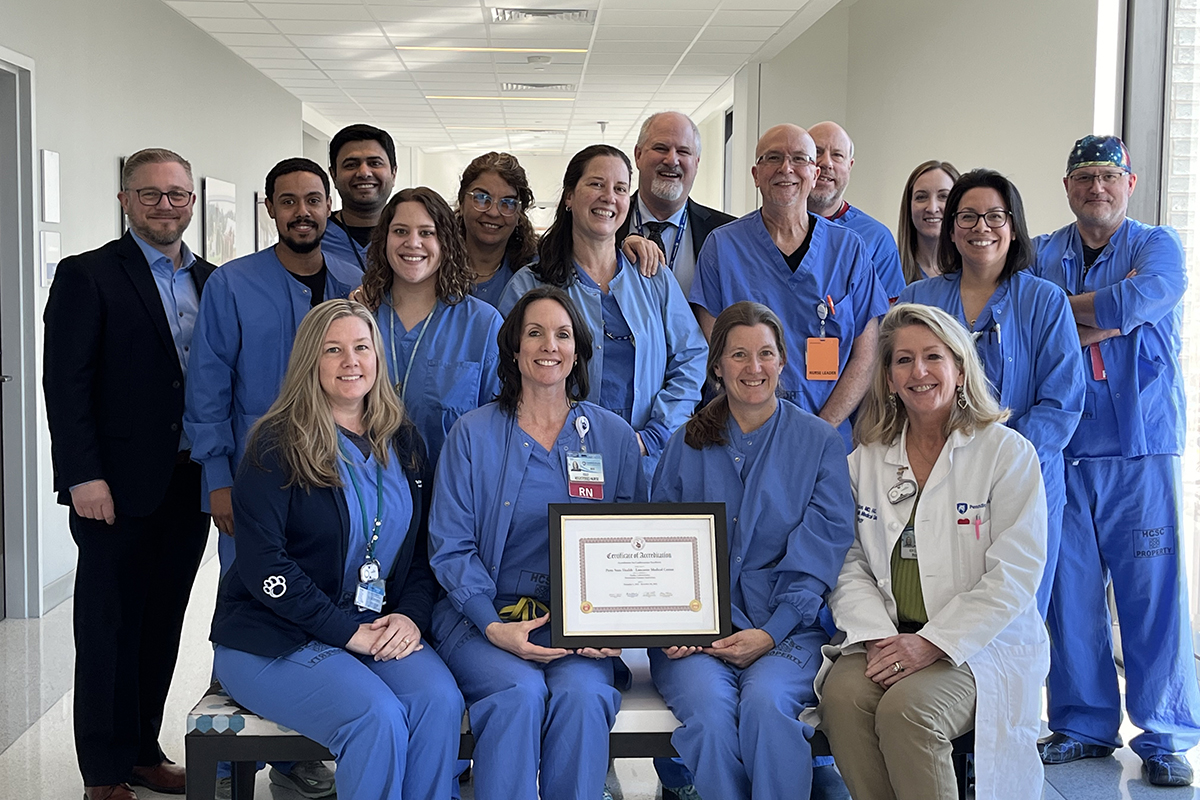In a bright and orderly healthcare facility hallway, a diverse group of professionals gathers for a celebratory photograph. The backdrop features pristine white and gray walls. The front row prominently displays four individuals, all beaming with pride, two of whom hold a black-framed certificate of accreditation. Among them, three women clad in blue scrubs sit beside a woman in tan pants and a green shirt, distinguishable by her white lab coat and a pen protruding from its pocket.

In the middle row stand five individuals—three women and two men—all varying in attire, including blue scrubs and casual wear. The back row comprises seven people, predominantly men, with two women included. Participants span various roles within the facility, from office workers to floor staff, and their name badges, necklaces, and lanyards are visible, adding a touch of personal flair. One notable attendee is dressed in a black suit, while another sports a bandana. Altogether, they represent a mix of ages and professions, unified in celebration and accomplishment.